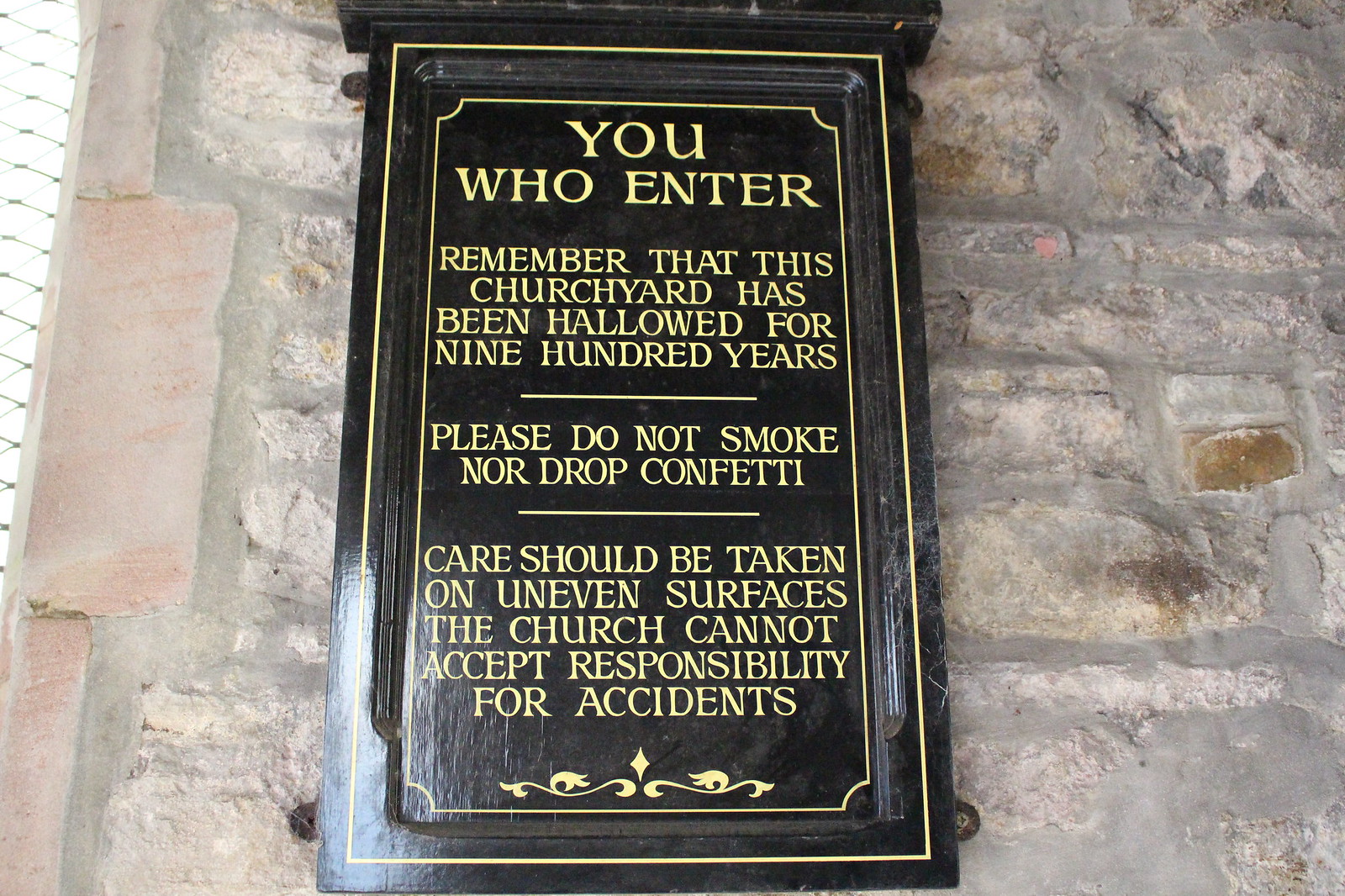This full-color photograph captures an aged stone wall, the gray stones speckled with patches of brown and red, hinting at centuries of weathering. Mounted on this wall is a distinctively framed black and yellow plaque, embodying a solemn message for visitors. The wooden plaque, edged in gold trim, reads in capitalized, yellow text: "You who enter, remember that this churchyard has been hallowed for 900 years. Please do not smoke nor drop confetti. Care should be taken on uneven surfaces. The church cannot accept responsibility for accidents." Horizontal yellow lines divide the text for emphasis. At the bottom of the plaque, a decorative spiral insignia adds a touch of elegance to the admonitory sign, reinforcing the historical significance and sacredness of the site.